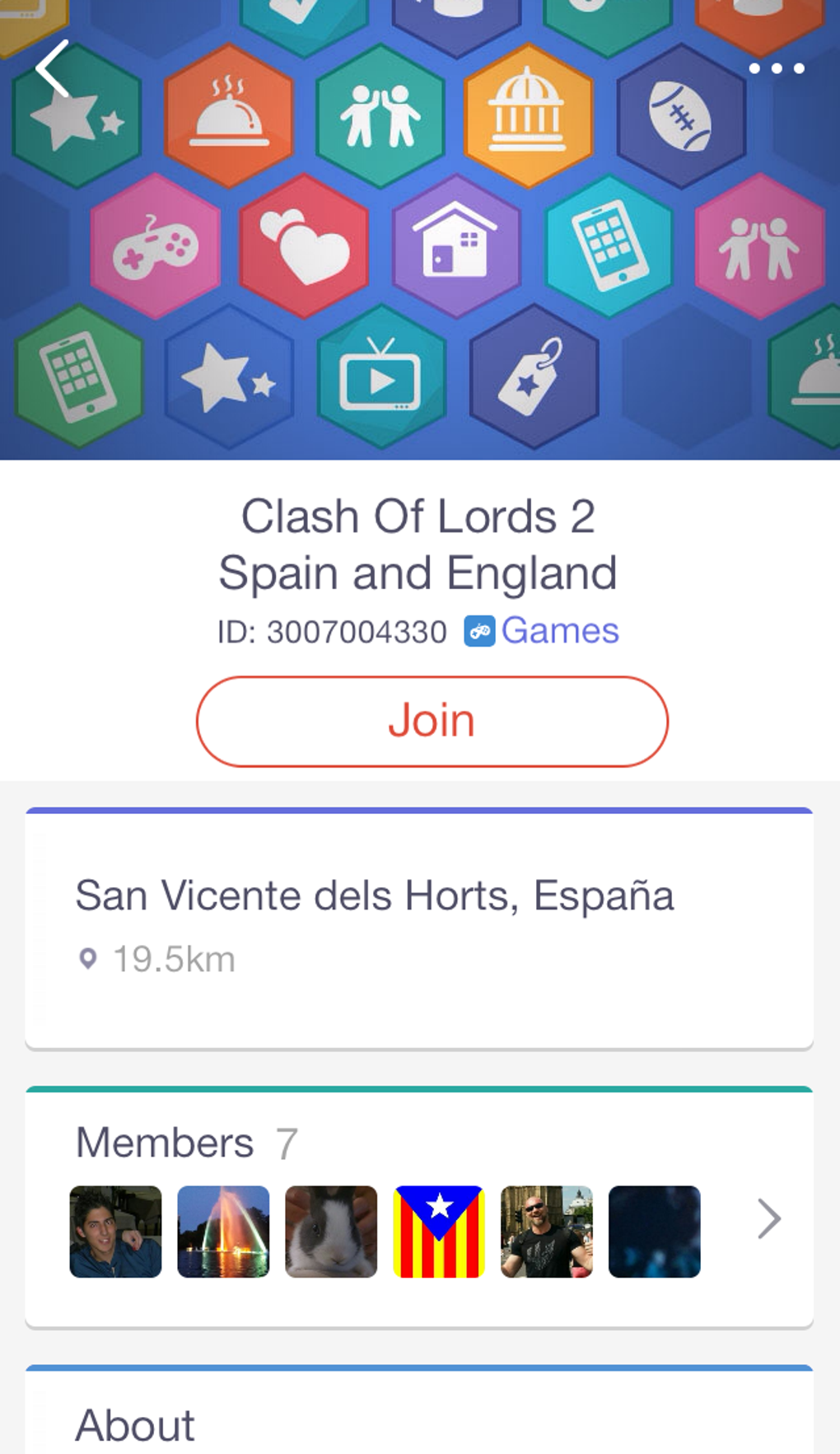A detailed screenshot reveals multiple elements on a white background, primarily featuring the game "Clash of Lords 2" associated with Spain and England, identifiable by the ID: 3007004330. The interface includes a blue square with a white video game controller symbol and a prominent red oval button marked "Join."

At the top of the screenshot, a collection of hexagons showcases various images: some depict video game controllers, others display hearts, stars, and a phone icon. On the left side of the screen, there's a back arrow, while the right side shows three horizontal dots, indicative of additional settings or options.

The location is specified as "San Vicente dels Horts, Hispana," accompanied by a location symbol and the distance of 19.5 KM. The group or community shown has 7 members and includes a visual array of six pictures:
1. The first picture features a man.
2. The second image appears to capture downtown lights, possibly reflected on a lake.
3. The third picture shows a predominantly white rabbit with grey markings around its eyes and ears.
4. The fourth image displays a flag with a blue downward-pointing triangle, a white star, and red and yellow stripes.
5. The fifth picture is of a muscular man.
6. The sixth and final image depicts what seems to be an array of bright lights.